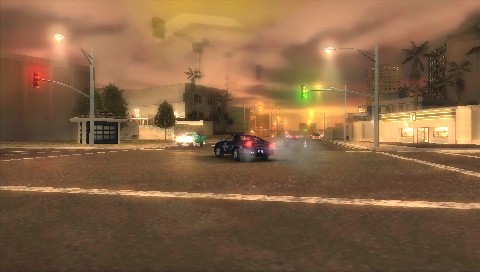The image features a vibrant but heavily blurred nighttime scene of a highway. In the midst of the motion, a black car is prominently veering off to the left. The right side of the highway is lined with low-rise buildings and a bus shelter-like structure, although its exact purpose is uncertain due to the setting likely being outside of England. Above these buildings, a green traffic light glows while a red traffic light is visible further left, signifying the divided directions of traffic.

In the background on the left, a tall building rises behind the blur of the traffic lights, adding an urban dimension to the scene. Street lamps contribute to the overall illumination, casting a disjointed glow on the surroundings. The sky is a murky hue, indicating the setting is nighttime. Further enriching the scene, palm trees can be spotted behind a wall on the right, suggesting a possibly warm, coastal location.